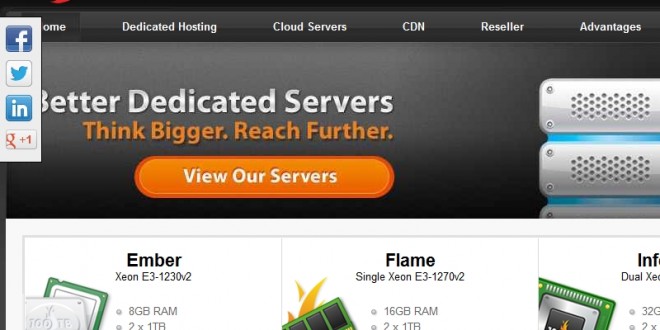This is a detailed screenshot of an e-commerce website specializing in the sale of dedicated servers. The top header features a gray background with prominent silver text that reads "Better Dedicated Servers." Directly beneath this, in striking orange text, it states "Think Bigger, Reach Further," accompanied by an orange call-to-action button that invites users to "View Our Servers." 

On the right side of this header section, there is a visually purposeful stack of white servers adorned with ventilation holes. Below the main header, the layout transitions into a product comparison chart set against a pristine white background, showcasing various server options. 

The first product listed is the "Ember Xeon E3 1230 V2," which is equipped with 8 gigabytes of RAM and dual 1-terabyte storage drives. Following this, the "Flame Single Xeon E3 1270 V2" is displayed, boasting 16 gigabytes of RAM, also with dual 1-terabyte storage drives. The third product is partially visible, characterized by a green casing and a central silver square, indicative of its premium design and build.

To the far left side of the screen, a vertically aligned tab features social media icons for Facebook, Twitter, LinkedIn, and Google Plus, suggesting various ways to share or follow the site. At the very top of the page, above the primary tagline, a set of navigational tabs can be found, labeled as "Dedicated Hosting," "Cloud Servers," "CDN," "Reseller," and "Advantages," providing quick access to other essential sections of the website.